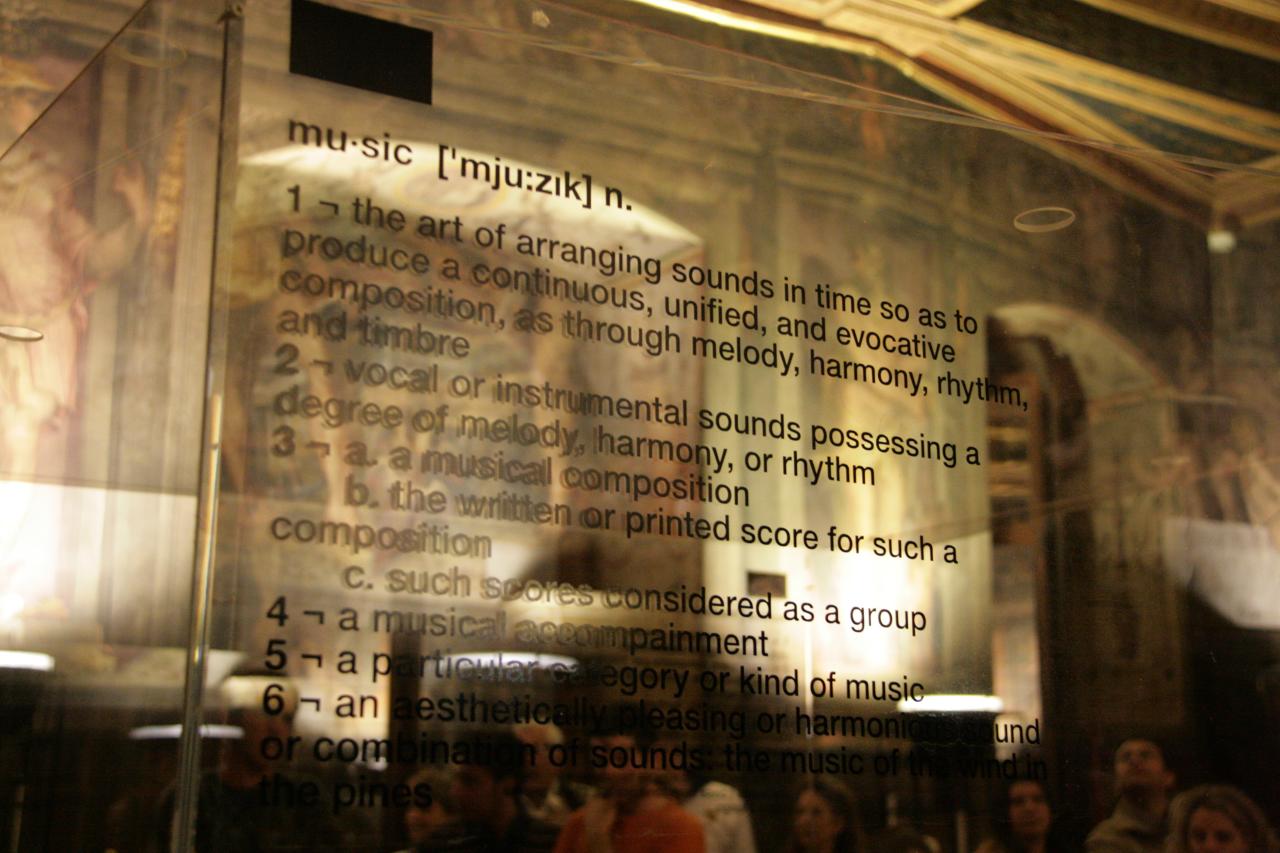The image displays a rectangular, beveled-edge plexiglass case or mirrored wall that presents the definition of 'music.' The text at the top spells out 'music' phonetically as "m-ju:zik" and identifies it as a noun. It proceeds to provide an extensive definition, divided into six parts. The first definition describes music as "the art of arranging sounds in time so as to produce a continuous, unified, and evocative composition as through melody, harmony, rhythm, and timbre." The second definition refers to "vocal or instrumental sounds possessing a degree of melody, harmony, or rhythm," while the third breaks down into sub-categories: a musical composition, its written or printed score, and such scores considered as a group. The fourth definition specifies "a musical accompaniment," and the fifth mentions "a particular category or kind of music." The sixth definition, which is partially obscured, hints at an aesthetically pleasing or harmonic sound. The plexiglass or mirrored surface reflects a background scene of people in a large, elegant hallway or music hall, glancing up towards the definitions.